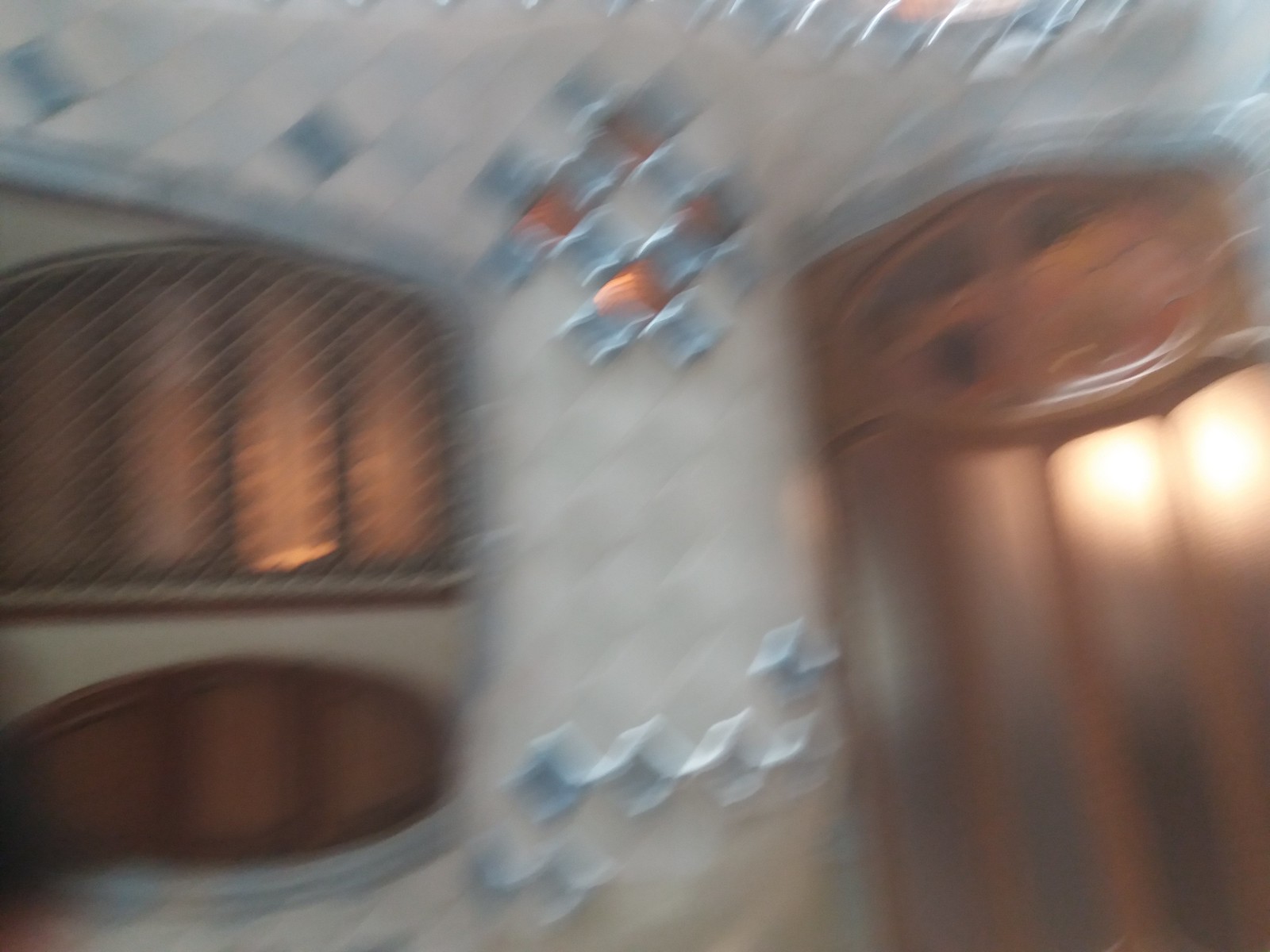This very blurry photo, likely taken accidentally while someone was in motion, captures a scene within an old building that exudes historical charm. The image features a prominent, large wooden oak door with bronze-colored, translucent glass windows, hinting at antique craftsmanship. Adjacent to the door is a window of similar design, topped with a grate. The structure, made from a mix of gray and rust-colored stones, creates a visually intriguing pattern that blends both order and randomness. The walls in the scene are adorned with small, pale gray checkered tiles, subtly contrasted against blue mosaic tiles that protrude slightly, adding a touch of texture. Scattered throughout the scene are rectangular and square shapes, some resembling terra-cotta and bronze-colored tile flooring. There are also a couple of gold, screen-like objects, which could possibly be small heaters or vents, adding to the building's aged and eclectic feel. The overall atmosphere suggests that this could be a European-style church or an ancient building, deeply embedded with historical and architectural significance.